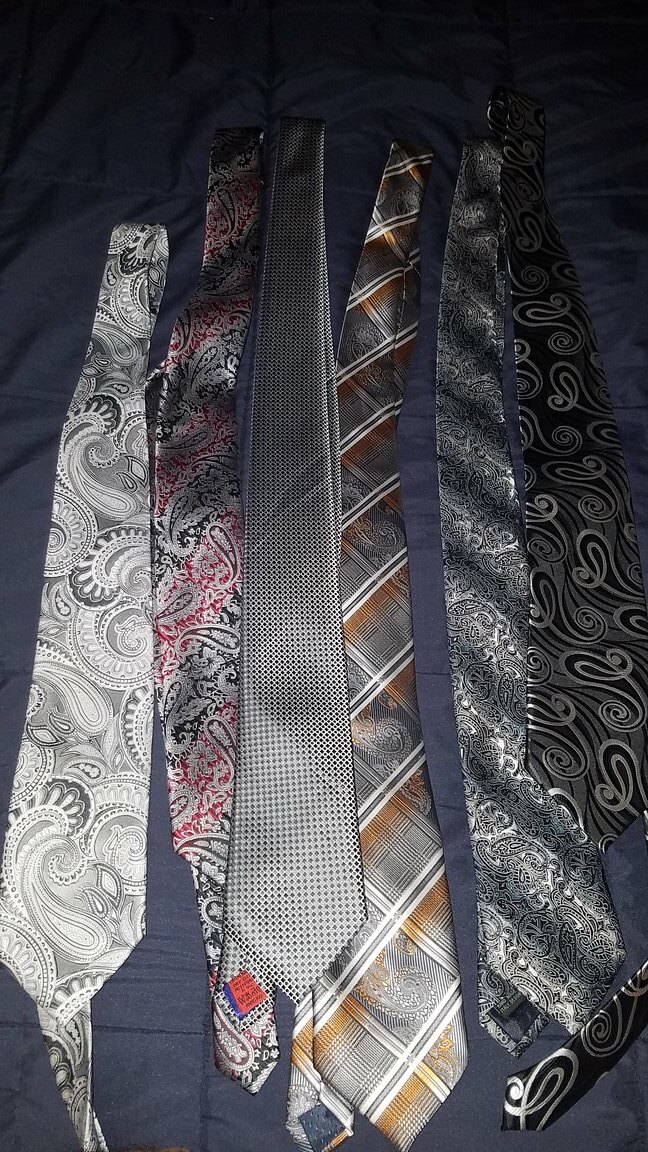The photograph showcases six ties neatly folded in half, aligned side by side on a blue blanket. Starting from the left, the first tie features a black and white paisley print. Next to it is a tie adorned with a black and red paisley pattern. The third tie is predominantly white, covered in a multitude of black dots. The fourth tie presents a checkerboard design intersected with white stripes, incorporating black and gold elements within the stripes. The fifth tie has an unidentifiable black and white pattern, possibly a fine houndstooth. Lastly, the rightmost tie displays another black and white paisley design. The ties rest on a blue blanket that has visible stitching at the bottom of the image. The photograph appears to have a darkened top section, contributing to a slightly dim ambiance.